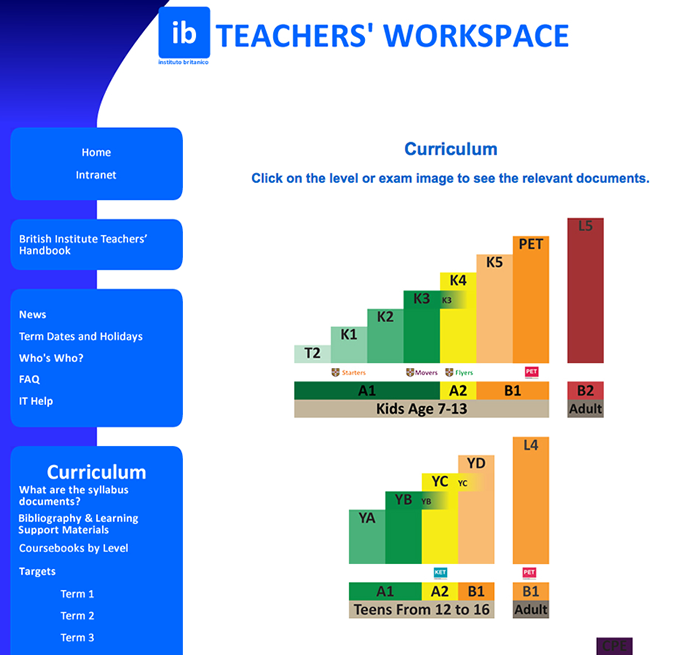The image depicts an educational dashboard titled "Teacher's Workspace" in bold blue text on a white background, with an "IB" logo at the top. Directly below this title, "Curriculum" is displayed, followed by a note stating, "Click on the level or exam image to see the relevant documents." The central area features two bar graphs stacked vertically. 

The upper bar graph includes categories such as T2, K1, K2, K3, K4, K5, PET, and L5. The bars vary in color: light green, dark green, yellow, light orange, dark orange, and dark red. The lower, shorter bar graph shows categories labeled YA, YB, YC, YD, and L4, with bars colored in green, yellow, light pink, and orange. These graphs illustrate different school grades, ranging from ages 7 to 13, teen categories from 12 to 16, and B2 adult levels.

To the left of the graphs, a navigation menu on a blue background with white text includes options such as Home, Internet, and British Institute Teacher's Handbook. Further options listed are Curriculum, What Other Syllabus Documents, Bibliography and Learning Support Materials, and Coursebooks by Levels. Additional entries include News, Terms, Dates, Holidays, and Who's Who.

Altogether, this image serves as a comprehensive digital workspace designed to streamline access to various curriculum documents and educational materials for teachers.